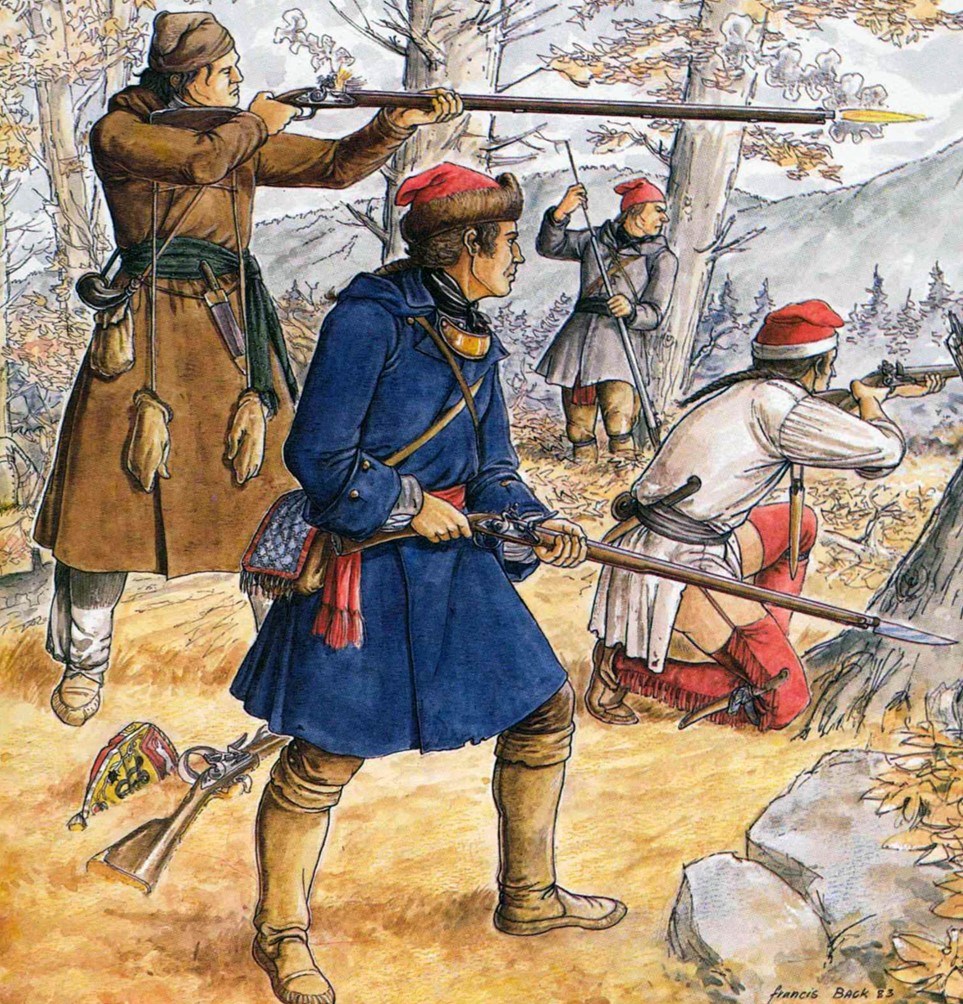The illustration depicts a detailed outdoor scene from the 1700s, featuring four light-skinned male soldiers amidst a forest with mountains in the background. Each soldier is dressed in period attire, including long coats in shades of blue, white, gray, and brown, camel-colored boots, and distinctive red and black hats resembling Christmas caps. They are equipped with muskets that have bayonets attached, and knives strapped around their waists and legs.

The composition of the soldiers shows two of them actively aiming and firing their muskets: one soldier in a brown coat on the left side has a yellow flame exiting his gun barrel, indicating he is currently shooting. Another soldier in a blue coat is in the process of cocking his gun while positioned with a bent knee, suggesting readiness to shoot. A third soldier in white with red fringe leggings and a red hat is kneeling, his gun aimed away but partially obscured. The fourth soldier hides behind a tree, peering around the trunk, seemingly waiting for the right moment to act. The setting is rich with natural elements, including various trees, gray rocks, and a straw or dirt-looking ground, all contributing to the historical and tactical atmosphere of the scene.